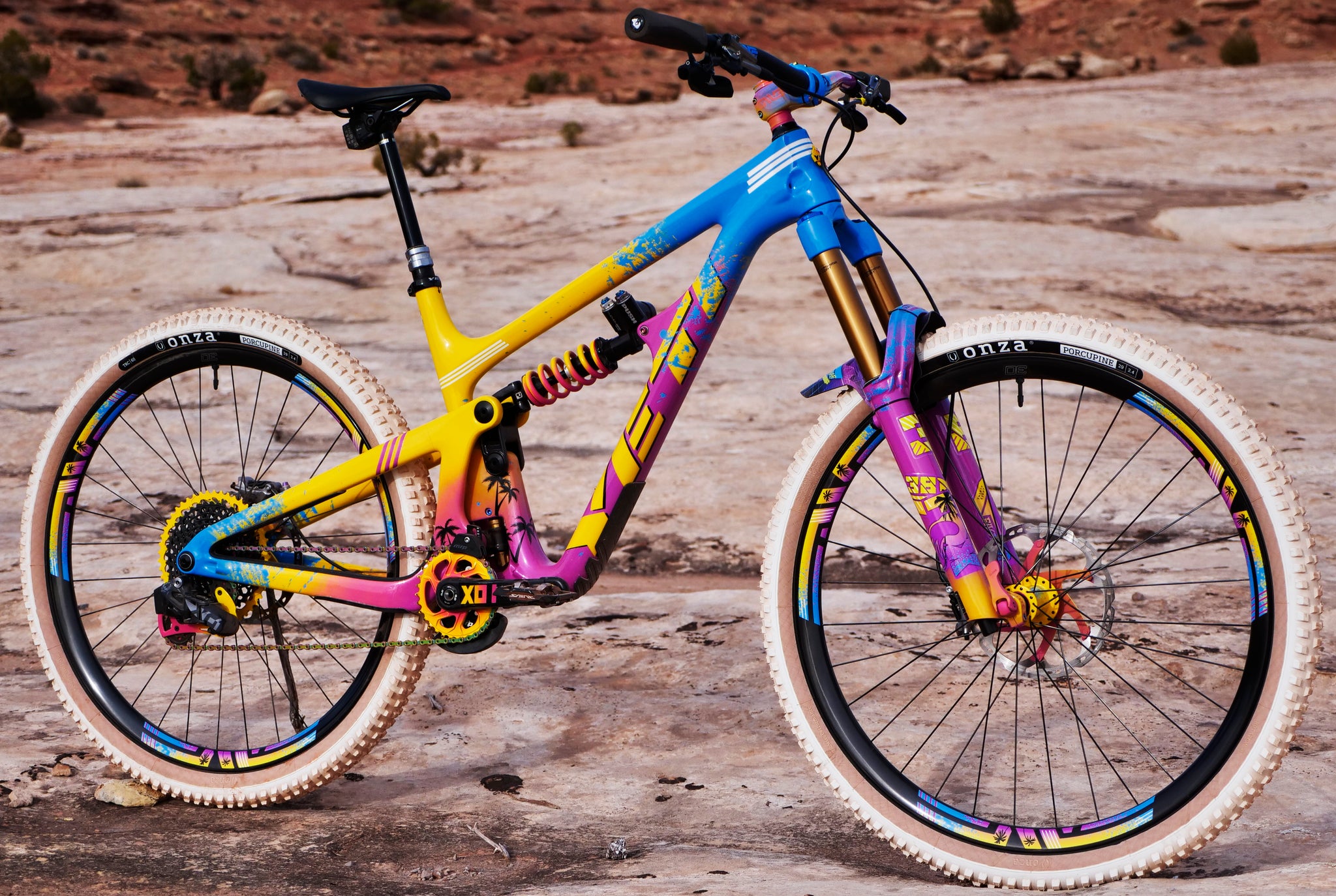The photograph features a vibrant kid's bicycle prominently positioned in a natural outdoor setting. The bike's frame is a lively combination of blue, yellow, and purple, adorned with decorative elements, including palm trees and the brand name "Yeti" in yellow letters sloping downward near the handlebars. The black handlebars and seat contrast with the colorful frame, and the seat appears to be elevated. The white-beige tires, marked with "Onza" (O-N-Z-A), and black rims stand out against the textured, grayish rock surface on which the bike rests. The chain is notably yellow, connecting to the bike's typical rear assembly. The background transitions into a higher elevation of reddish rocks, with a mix of dark beige, brown, and darker brown tones, suggesting a southwestern landscape. A few bushes can be seen scattered among the loose rocks in this expansive, natural dirt area. The bike, oriented towards the right, dominates the image, while the varied terrain enhances the overall rugged and adventurous feel of the scene.